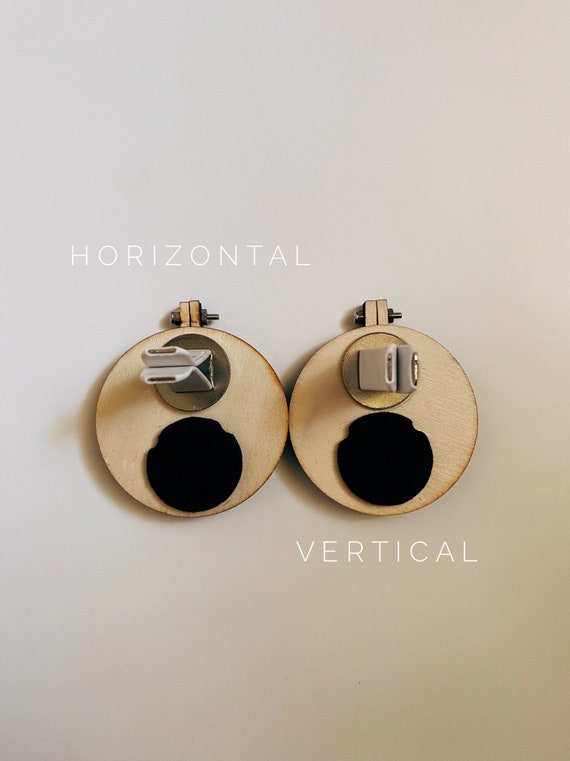This is a rectangular photograph approximately six inches high by four inches wide, featuring a gradient background transitioning from light gray at the upper left to light tan and into regular brown at the lower right. The image prominently displays two wooden, round objects positioned side by side, each adorned with a metal clip at the top, secured by a screw running horizontally through them. These screws seem to tighten or loosen the clips that may connect to other components. Above the left object, white text reads "horizontal," while below the right object, similar white text reads "vertical." Each wooden circle also has a smaller black circle beneath it, accompanied by a small, gray, plastic double-prong component perched above. The entire setup suggests some kind of mechanical or electronic functionality, possibly involving an electrical connection given the white plug that could accommodate a computer wire. The background provides a visually pleasing ombre effect against which these intricate components are set.